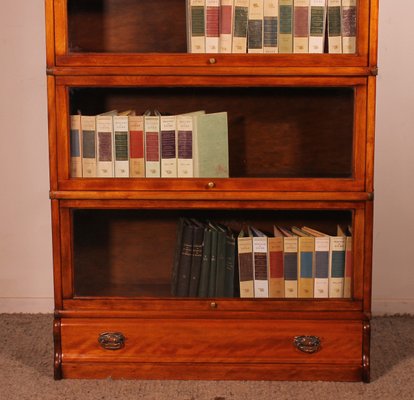The central focus of the image is a dark wooden chest, positioned against a light pink wall and above a brown floor. This chest comprises three shelves and a bottom pull-out drawer adorned with two sleek metal handles. Each shelf contains various books, binders, and folders arranged in a distinct pattern: the top shelf has items predominantly shifted to the right, the middle shelf to the left, and the bottom shelf to the right again. The collection includes multicolored labels on the binders and books with spines in hues of green, red, purple, and blue. Among the items, black-colored folders are noticeable on the bottom shelf, particularly in the middle section.